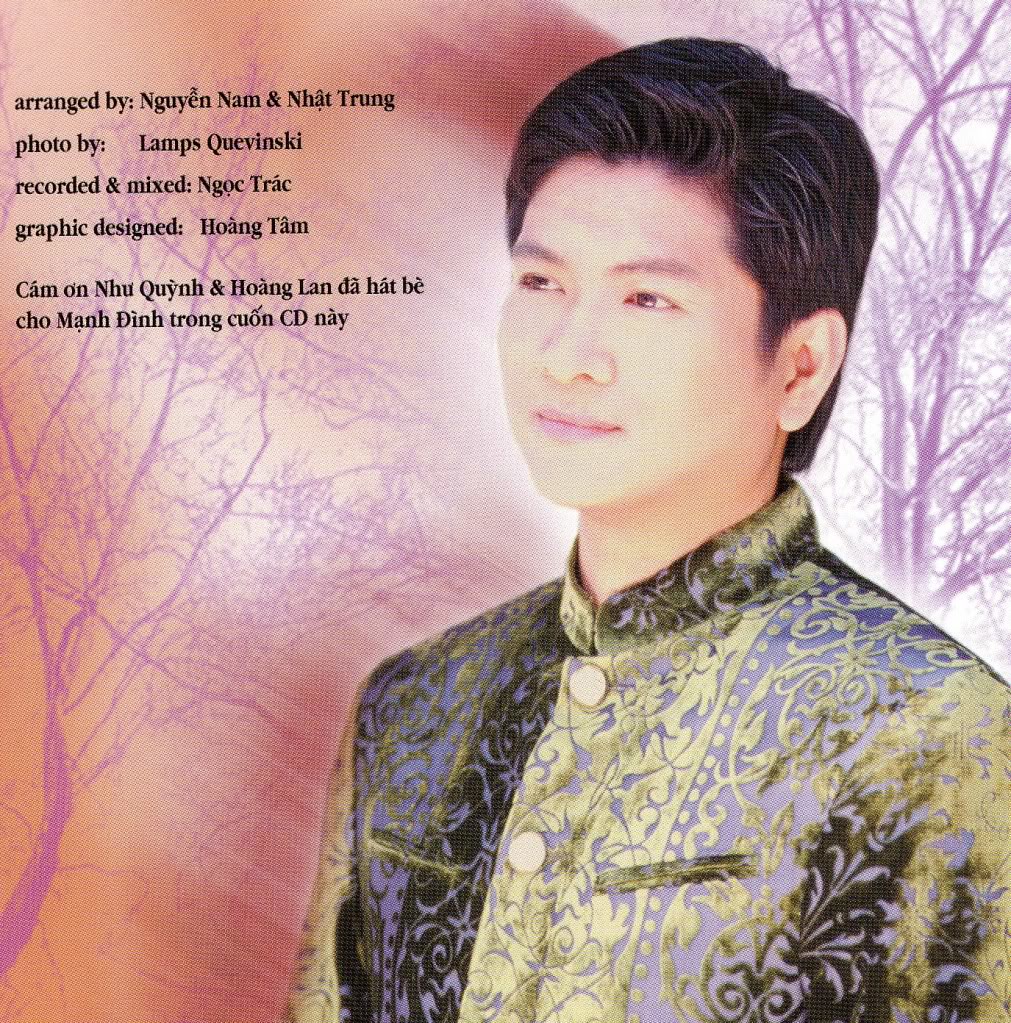The image is a slightly taller-than-wide, yet nearly square-shaped photo, likely representing the back cover of a CD. Prominently featured on the right side is the upper half of an Asian man, appearing to be in his late 20s or early 30s. He has straight, short black hair, parted at the side with bangs styled upward, and he is gazing towards the upper left corner with a slight smile. The man's ears are exposed, and he has brown eyes. His attire is a button-up, high-neck silk shirt in green with light blue stripes, adorned with intricate scrolling designs of leaves and vines.

The background of the image transitions from white in the upper right corner to shades of orange and red to the left, overlaid with thin, pale purple trees. In the upper left-hand corner, black text states: "Arranged by Nguyen Nam and Ngoc Truong. Photo by Lamps Kavinsky. Recorded and mixed at NGOC TRAC. Graphic design by Hoang Tam. Cam Anh Nhu Khoi and Hoang Lan Da Hat Bay. Chau Man Dinh Truong Kwan. CD Nay."